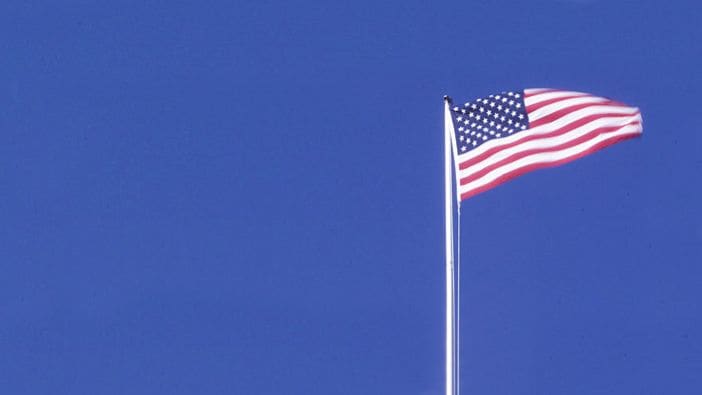The image captures a somewhat low-resolution, slightly blurry still frame that appears to be shot from the ground looking up. Dominating the background is a deep sky blue that extends almost uniformly across the frame, creating a serene backdrop. On the right side of the image stands a tall flagpole that reaches approximately two-thirds up from the bottom. Attached to this flagpole and fluttering towards the right edge of the frame is the American flag. The flag, vividly detailed with 50 white stars on a blue canton and 13 alternating red and white horizontal stripes, is seen clearly with a cord fastening it to the pole. The flag appears to be catching the wind, which gives it a dynamic feel, almost as though it is reaching out towards the right side of the image. The lighting suggests that the sunlight may be coming from the left, highlighted subtly by the reflection seen along the pole. The composition beautifully contrasts the flag's vibrant colors against a seamless, expansive blue sky, emphasizing its patriotic symbolism.